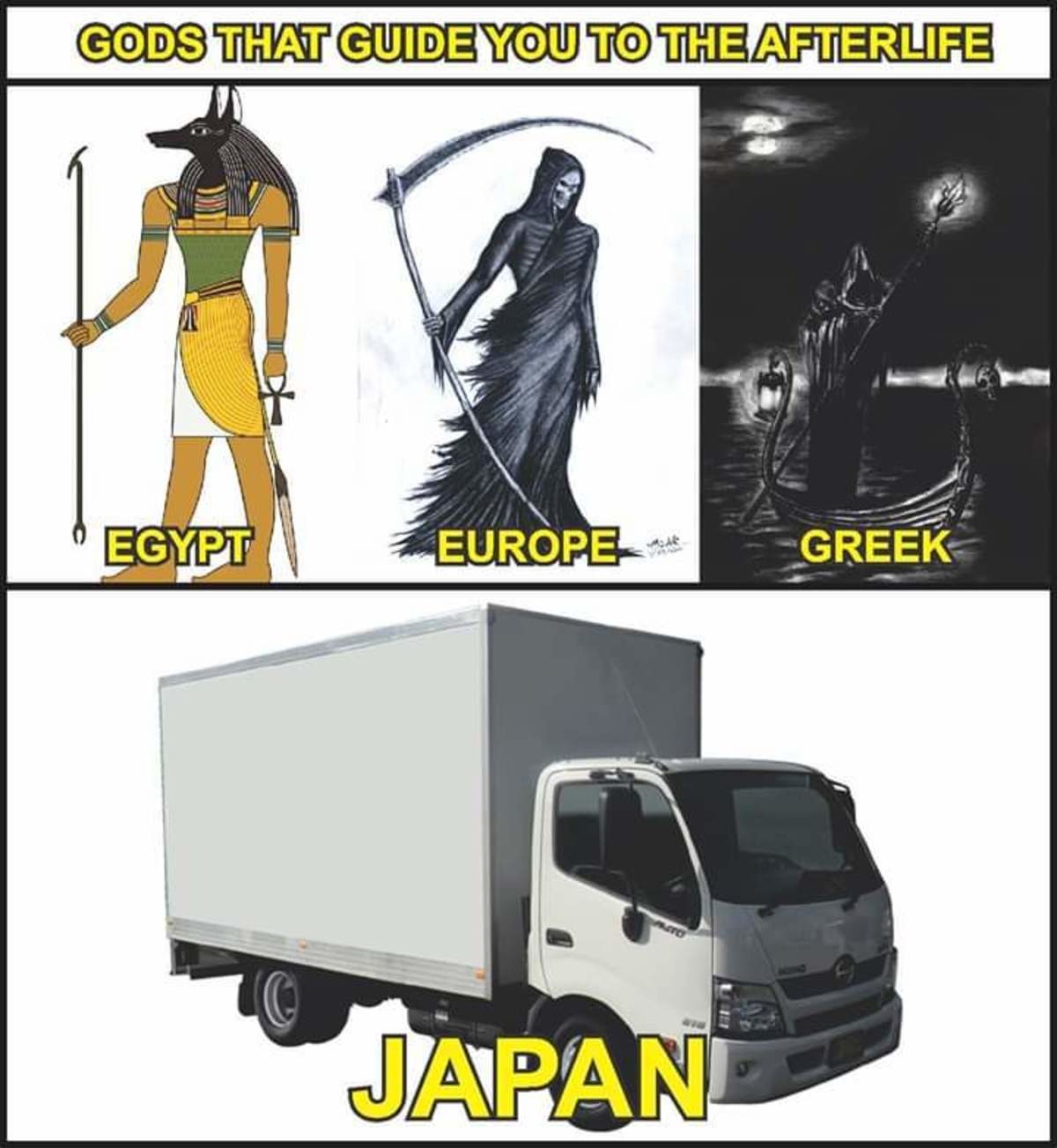The image features a white background bordered in black and is divided into sections with black outlines. At the top, yellow text with a black outline reads, "Gods that guide you to the afterlife." Below this heading, three images are displayed from left to right. The first image, labeled "Egypt," depicts the Egyptian God Anubis, characterized by his tan skin, dog head, and multi-colored attire including blue wristbands, a green shirt, and a yellow and white skirt. He holds a black ankh in one hand and a white-and-black staff in the other. The second image, labeled "Europe," features a grim reaper dressed in a tattered black cloak with a visible skeleton and a long black sickle. The third image, labeled "Greek," shows Charon, the mythological ferryman, standing on a boat in a dark sea, holding a lantern. The sky behind him is black with a white moon. At the bottom of the image, another section contains the label "Japan" in yellow text outlined in black, beneath which is a white box truck with black tires and tinted windows.